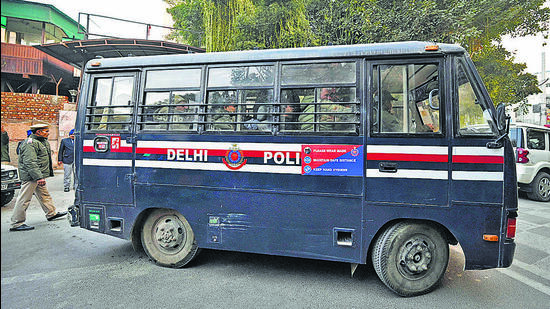This photo captures a vintage navy blue bus associated with the New Delhi Police Department. The bus, which has a squarish and slightly old appearance, features a distinct set of stripes—white, red, dark blue, and another white stripe—running horizontally across the middle just below the windows. It bears the inscription "DELHI POLI" in white letters, though part of the word is obscured by a small red and blue sticker or sign. The bus windows are fitted with bars, hinting at a secure transport, possibly for personnel who appear to be dressed in military or olive-green attire. 

The scene unfolds on a city street during the daytime. The bus is parked, revealing its dirty black wheels and a single visible side mirror. Situated directly behind the bus is a man donning a green jacket, khaki pants, and running shoes. Adjacent to this setup is a white SUV or another type of vehicle, and both are flanked by trees and a building to the left. Additionally, a brick building with a green canopy is visible in the background, enhancing the urban atmosphere of the image.